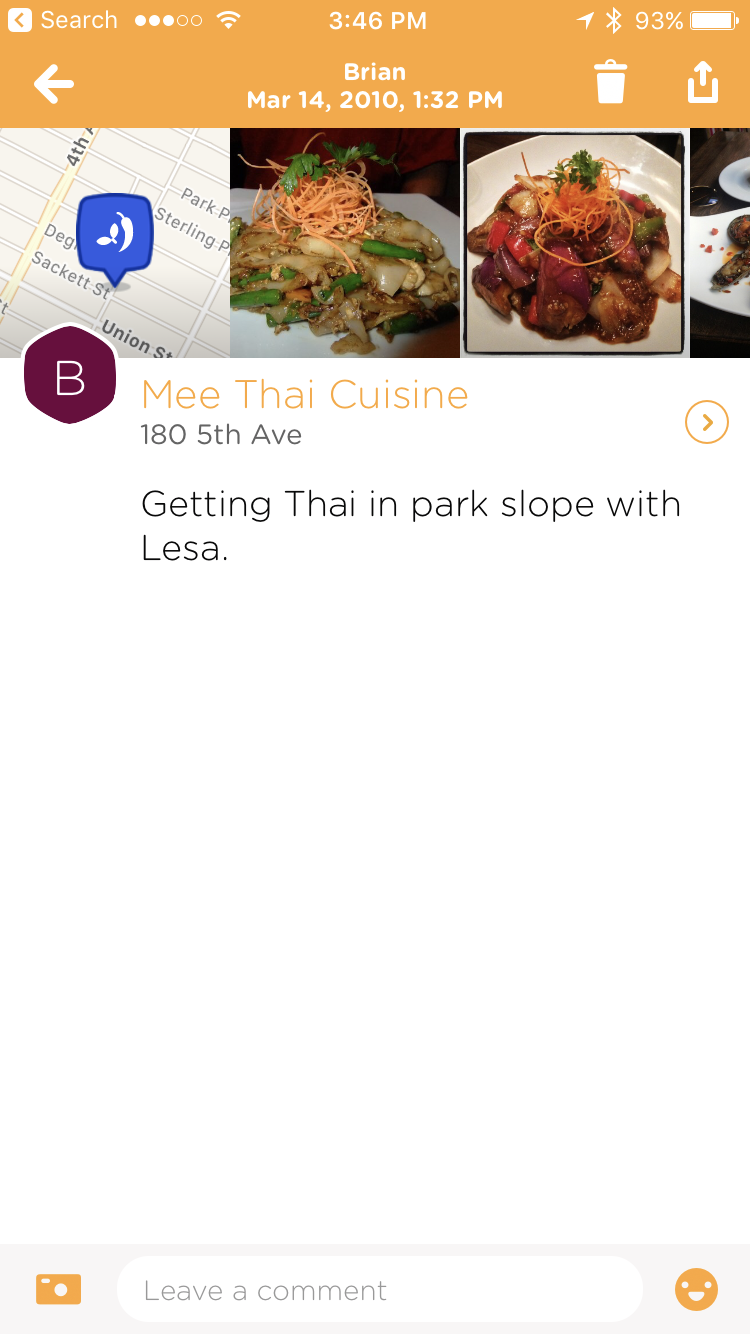A smartphone screen is shown with a mix of interface elements and a gallery of photos. At the very top left, there's a search bar alongside a back arrow inside a white box. Next to it, there are five signal strength circles, three of which are filled, indicating a moderate connection. Adjacent to this, the WiFi symbol displays that the device is connected. The time reads 3:46 PM, and on the right side of the status bar, there's another icon and the number 93%, signifying the nearly full battery.

Below this status bar, the name "Brian" is centrally located, followed by a timestamp "March 14, 2010, 1:32 PM". Further to the right, there's a trash can icon and a download button symbolized by a 'U' with an upward-pointing arrow in the middle.

Four photos are displayed below this section. The first image appears to be a map with an arrow pointing to a location marked by a pepper icon. The second and third images are food dishes presented in square frames. The fourth image is a partially visible plate featuring more food.

Beneath the first image, a letter 'B' in brown is visible, followed by the text "_me Thai Cuisine_" and an arrow inside a yellow circle. Below the gallery, there's the text "185th Avenue" and the sentence "Getting Thai in Park Slope with Lisa." These details together paint a picture of someone documenting a visit to a Thai restaurant, capturing specific interface details and snapshots of the meal.